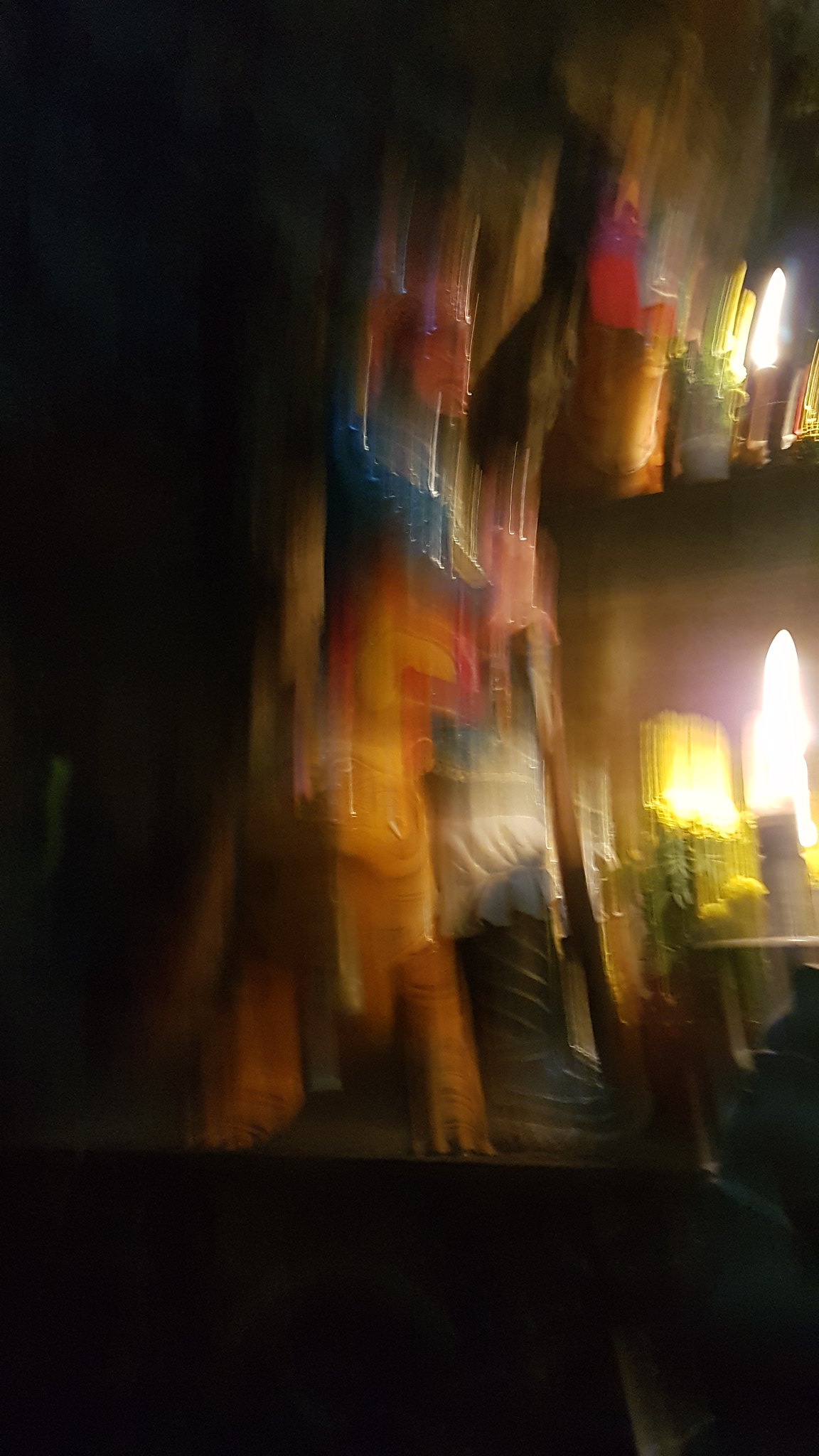The photograph captures a dynamic and blurred scene, as if the camera was in motion when the picture was taken. On the left side of the image, a deep, impenetrable blackness dominates, creating a stark contrast with the rest of the composition. In the center, vague shapes suggest the form of a person, possibly standing still and observing something beyond the frame. To the right, a row of distinctly different lamps are displayed, each with unique and imaginative shades that seem to be part of a store window display. One lamp features a shade resembling a yellow cob of corn, while another boasts a design that looks like a projectile or rocket. Despite the overall blur, the peculiar assortment of lighting fixtures on a shelf hints at a whimsical and eclectic collection. This image, though unclear and chaotic, intriguingly invites the viewer to imagine the scene as one of peculiar observation through a shop window full of creative and varied lamps.